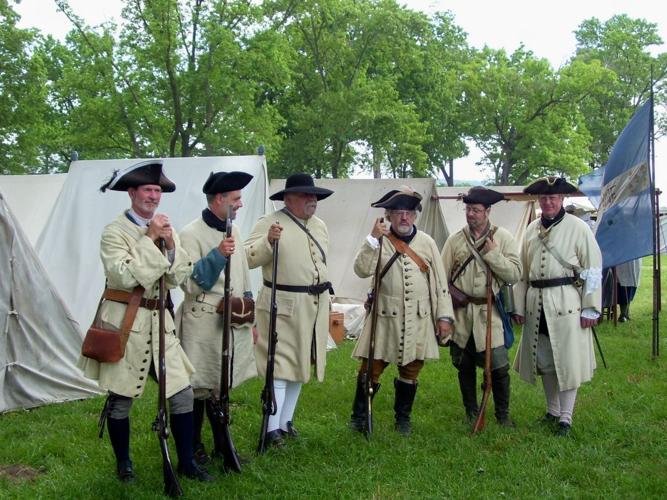A realistic, horizontally-oriented color photograph depicts six men standing on a lush green lawn with verdant trees in the background under a whitish daytime sky. Dressed in historical attire evocative of colonial European or American times, the men appear to be participants in a historical reenactment, possibly from the Revolutionary War era. Five of the men wear black felt tricorn hats while one sports a black brimmed hat. They are clad in beige frocks, white thigh-length coats with multiple buttons, black boots, various leggings, and stockings. Each man holds a wooden musket, except for one who carries a saber in his belt. The backdrop features white cloth tents typical of historical encampments and a partially unfurled blue and white flag. All six men pose facing the camera, their expressions set against the vivid historical setting.